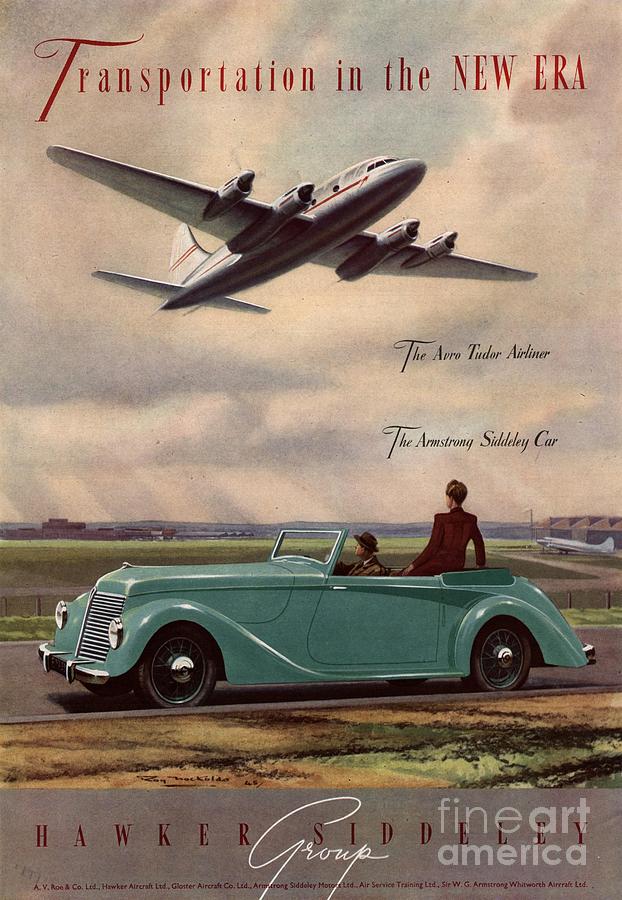The poster, seemingly set in the 1940s, prominently features the bold red text "Transportation in the New Era" at the top. The focal point is a beautifully detailed turquoise convertible car, accentuated by its vintage design. Inside the car, which appears to be parked possibly on airport grounds, sits a man in the driver's seat and a woman perched on the back seat, both gazing upward. Above them soars a modern aircraft, symbolizing the juxtaposition of past and future transportation. The bottom of the poster bears an inscription by the producer, reading, albeit partially obscured, "Hawker, possibly Sydney," followed by the clear notation "Fine Art America." The scene masterfully captures the transition from classic to contemporary travel, merging old-world charm with futuristic aspirations.